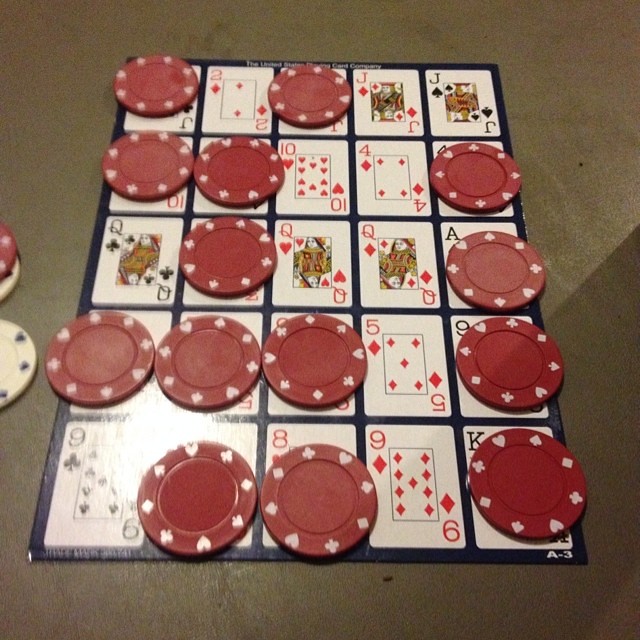This photograph depicts a detailed scene captured at an angle, showcasing a tabletop surface made of dark gray wood. Dominating the table is a grid-like structure, possibly made of cardboard or black plastic, marked at the bottom right with "A-3." The grid itself is composed of playing cards arranged in a 5x5 configuration, separated by black lines. Each row contains five cards, beginning with the top row which showcases: the Jack of Clubs, the Two of Diamonds, the Jack of Hearts, the Jack of Diamonds, and the Jack of Spades. 

Interspersed across several of these cards are red chips bearing white symbols representing the suits of clubs, hearts, diamonds, and spades. Each chip features these emblems encircling their perimeter. Eight of these chips are visible, adding a layer of complexity and intrigue to the arrangement. The contrast between the vibrant red chips and the monochromatic tones of the cards and grid enhance the intricate and strategic nature of what appears to be a game or puzzle setup.